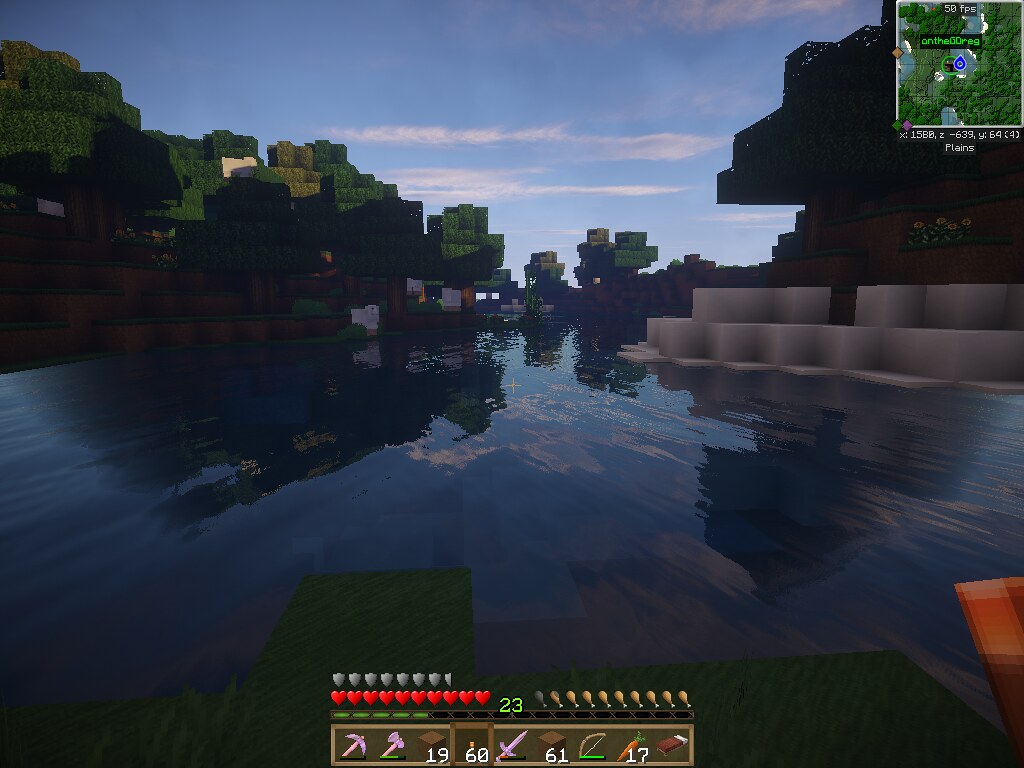This screenshot from the popular block-based video game Minecraft captures a serene and tranquil landscape in the game's unique pixelated style. The scene appears to be set in early morning or late evening, as suggested by the soft, warm lighting and elongated shadows. In the foreground, vibrant greenery and dense foliage dominate, with cube-like trees characteristic of Minecraft, featuring dark green leaves and sturdy brown trunks. The landscape gently descends towards a calm and reflective body of water located in the middle portion of the image. The water's surface mirrors the sky and surrounding trees, albeit with a slightly distorted reflection, enhancing the peaceful ambiance of the setting. The overall composition and lighting imbue the scene with a sense of quiet solitude and natural beauty.